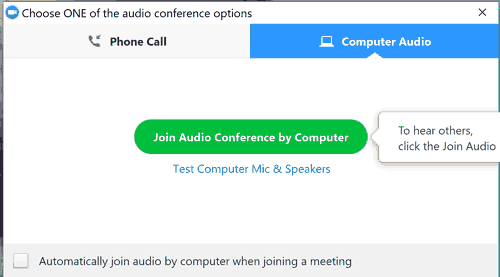This image is a screenshot capturing a Zoom call interface, specifically focusing on the audio conference options menu. The blue Zoom icon with a white camera logo is prominently displayed in the upper-left corner, indicating the platform. To the right of the icon, there's a label reading "CHOOSE ONE OF THE AUDIO CONFERENCE OPTIONS" in uppercase text.

Below this, two rectangular buttons offer different audio connection methods. The left button, labeled "Phone Call," features an icon of a phone with an arrow pointing toward it. This button has a gray background, signifying that it is not selected. The right button, labeled "Computer Audio," displays an icon of a laptop. This button has white text on a blue background, with a small white triangle at the bottom center, showing that it is currently selected.

Centered on the screen is a green action button with white text that reads "Join Audio Conference By Computer." To its right, there is a white pop-up message advising, "To hear others, click Join Audio." Below the green action button, there's a blue text link that reads "Test Computer Mic & Speakers." 

At the bottom of the interface, there's an unchecked checkbox next to the text, "Automatically join audio by computer when joining a meeting." The background of this checkbox section is light gray, while the central area of the menu is solid white. In the upper-right corner of the screen, there is a small "X" icon to close this pop-up menu.